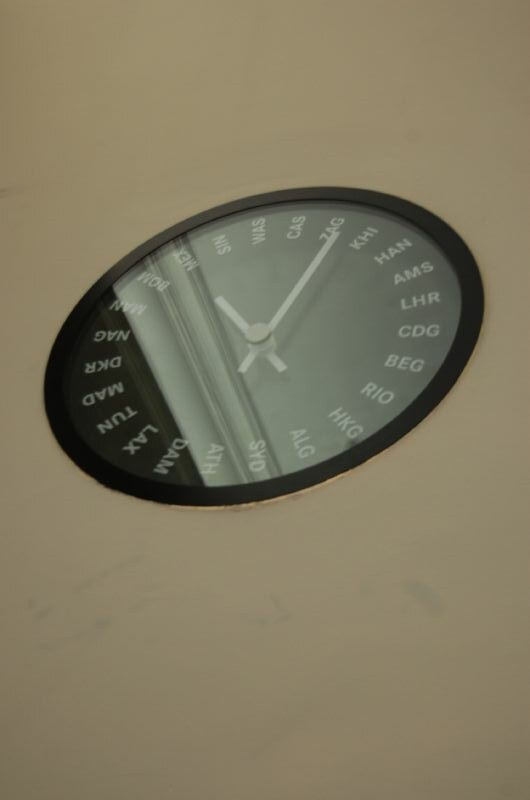This photograph captures a uniquely designed wall clock with a round shape, enclosed in a sleek black frame. The clock face features a sophisticated dark gray background adorned with light gray markings, including hands and inscriptions. Notably absent of traditional numbers, the face is punctuated by various three-letter acronyms such as ZAG, KHI, HAN, AMS, and LHR, arrayed thoughtfully around its circumference.

The clock is mounted on a wall painted in a warm light brown hue, contributing to the cozy yet professional atmosphere that suggests the setting is within an office building. Reflections on the clock's surface indicate white ceiling moldings, adding to the room's refined aesthetic. The photograph is taken from a low angle, offering an upward perspective that accentuates the clock's position and interaction with its surroundings.